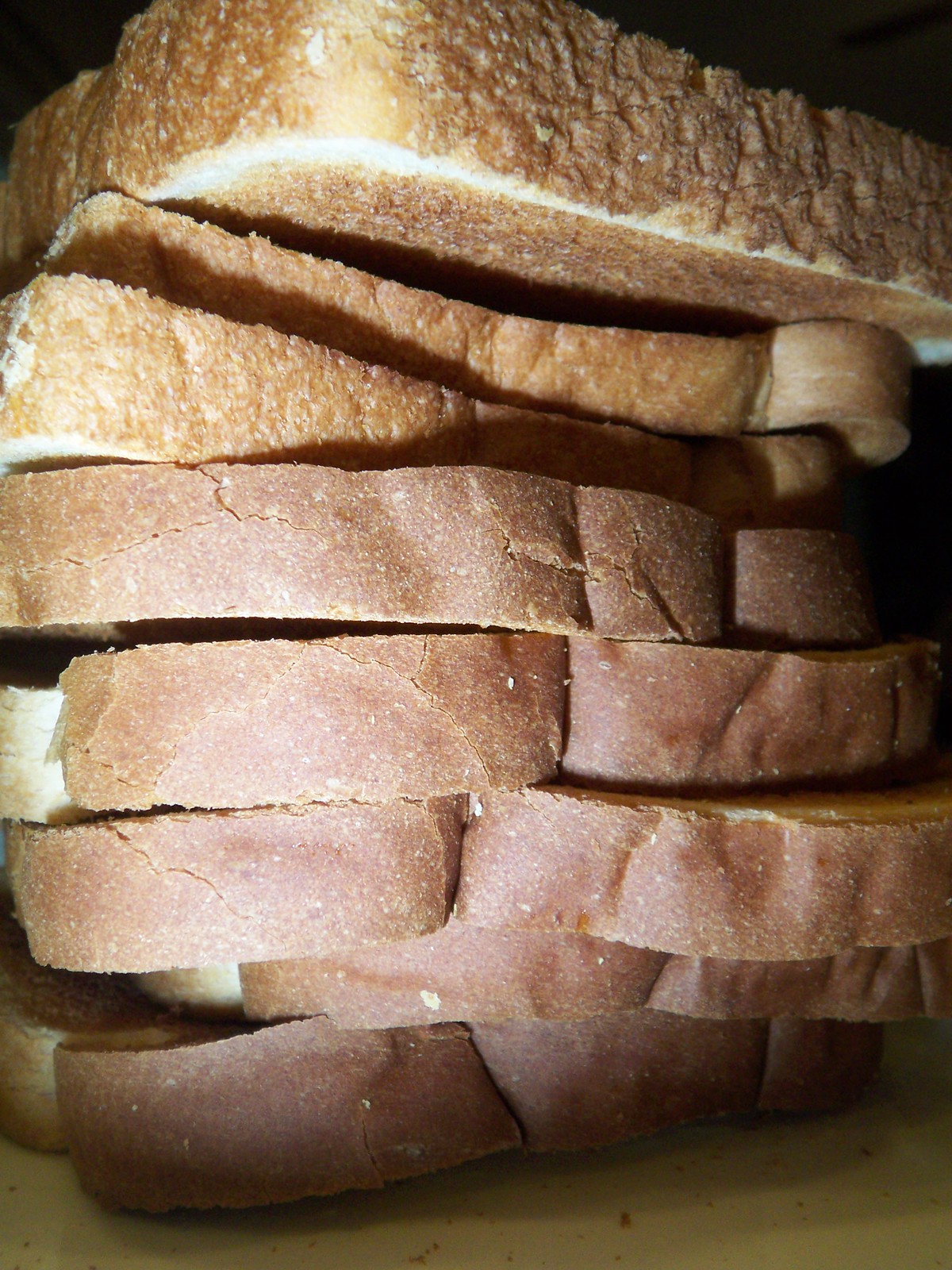In a photograph set against a completely black background, eight slices of American white bread are stacked haphazardly on what appears to be a yellowish board. The bread, featuring a brown crust, ranges in thickness and uniformity. The bottom slices are uniform, likely store-bought, with a lighter inner color, while the top three pieces seem irregularly cut, suggesting they might be homemade. The topmost slice appears toasted and browned around the edges, with visible butter suggesting it was fried. Soft crumbs are scattered at the bottom, and bright light illuminates the bread, highlighting its texture and irregular stack.